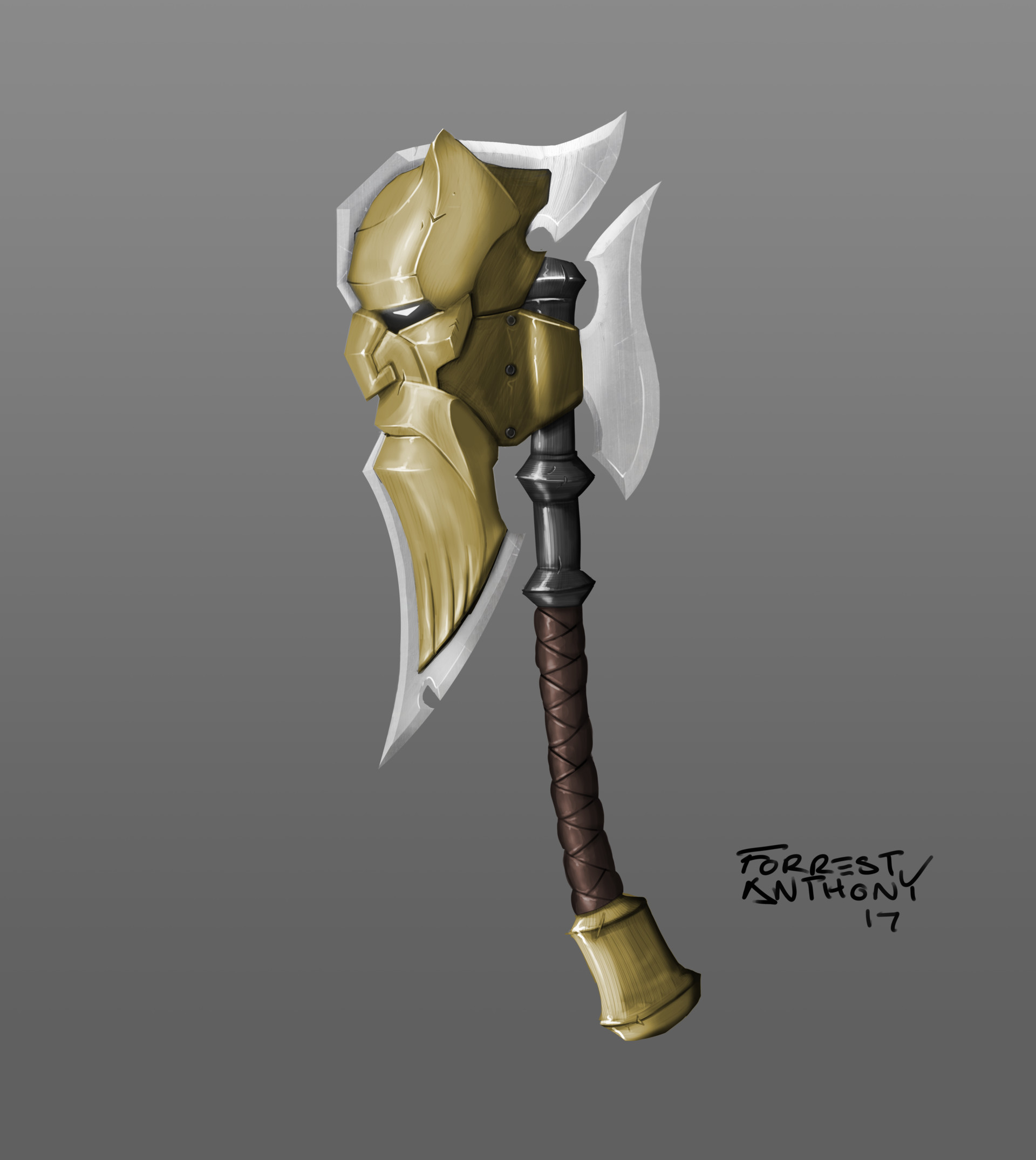This image depicts a detailed artwork of an axe centered against a matte blue-gray background, reminiscent of a painting. The rectangular image, approximately six inches high and four inches wide, features an axe that stands three to four inches tall. The base of the handle is a golden bell shape, transitioning into a brown corded wrap for about an inch. The upper part of the handle is dark brown to black, with metallic gray accents and two protruding knobs.

The axe head itself showcases an intricate side profile of a man's face, adorned with a golden cowl, featuring a hooked nose and pointed beard. His eyes are represented with deep black and white elements, while a prominent silver blade runs vertically across his face from nose to the top, with another almost touching blade on the reverse side. In the lower right corner of the image, the artist’s name "Forrest Anthony" and the year "17" are inscribed in black.